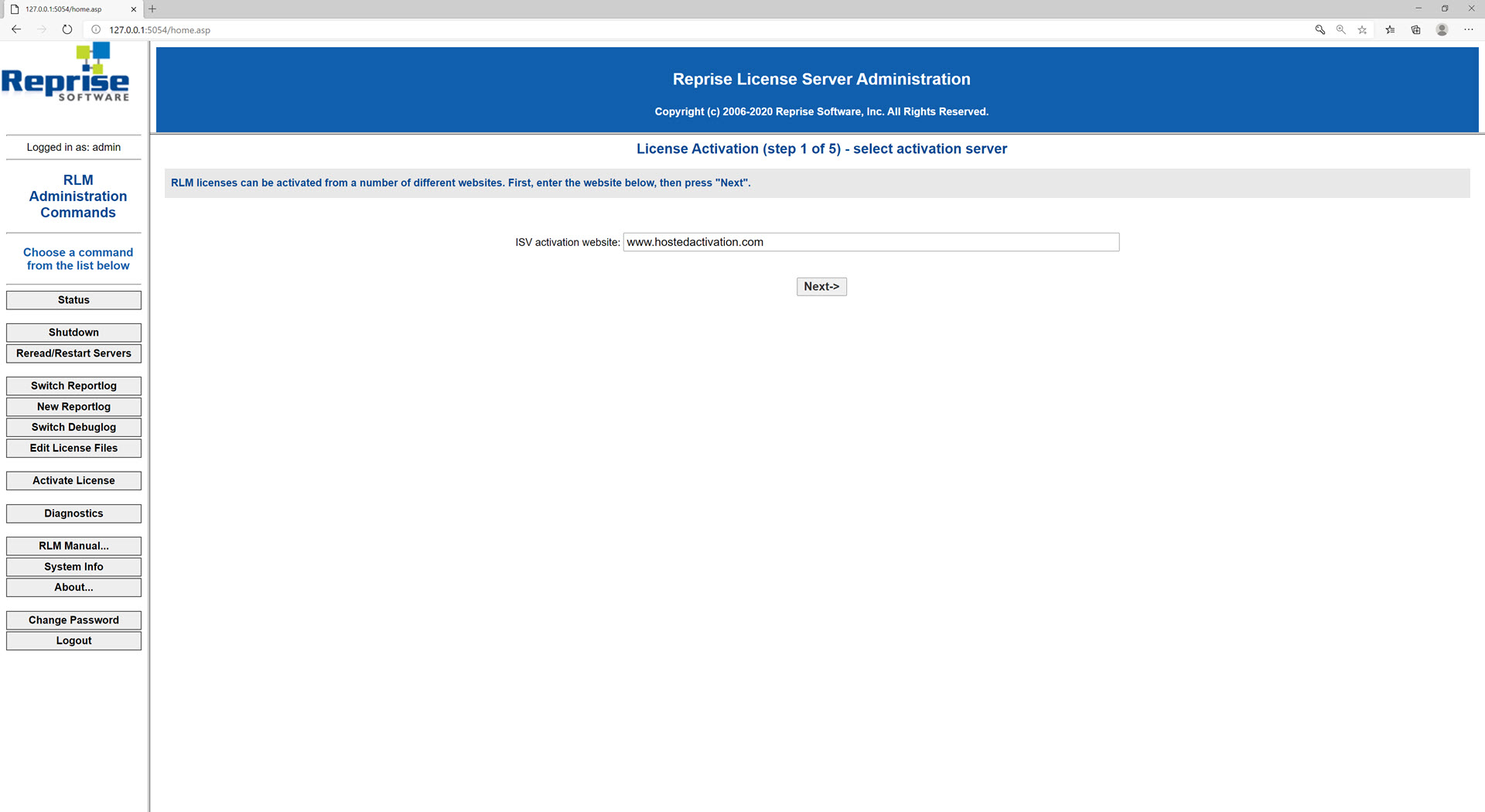This screenshot, depicted in landscape orientation, captures a full webpage interface from a software management site.

In the top left corner, there is a partially obscured text, roughly "127.00", extending to the right edge in grey, ending with an "X" button to close the window. The next row features a back arrow, followed by the repeated text "127.00.1.5". On the far right, there are some indistinguishable icons.

On the left side, there is a vertical navigation column which begins with the heading "Reprise Software", followed by "Logged in as Admin", and a list titled "RLM Administration Commands". The list includes options such as: Status, Shutdown, Reread, Restart Servers, Switch Report Log, New Report Log, Switch Debug Log, Edit License Files, Update License, Diagnostics, RLM Manual, System Info, About, Change Password, and Logout. This column is separated from the main content area by a grey line.

The main content area starts with a broad blue stripe displaying the text "Reprise License Server Administration, Copyright 2006-2020, Reprise Software, Inc., All Rights Reserved". Below this, on a blue and white background, the section reads "License Activation, Step 1 of 5, Select Activation Server", followed by a grey stripe. Instructions are provided: "RLM licenses can be activated from a number of different websites. First, enter the website below, then press Next". The input field is labeled "ISV Activation Website" with the placeholder "HostedActivation.com". At the bottom, there is a "Next" button to proceed.